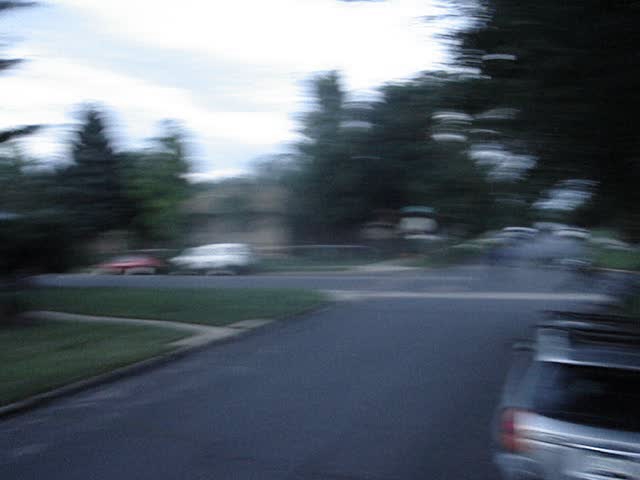The image depicts a blurry urban street corner scene. On the left side, there is a front yard featuring a sidewalk that seemingly leads somewhere, partially obscured by a tree. Adjacent to this yard, a cross street stretches horizontally across the picture. Parked on this cross street are a red car and a white car. Beyond these vehicles, there is a brown house, possibly constructed with bricks, with trees dotting its front yard. 

Moving towards the right, two cars are parked either in a driveway or a side yard adjacent to the house. The primary street extends upward from the bottom of the image alongside this house. Although it is difficult to determine if there are additional cars on the street due to the blurriness, numerous trees populate the background, adding a lush, green backdrop. Finally, in the bottom right corner, a silver SUV is visible, completing the scene.